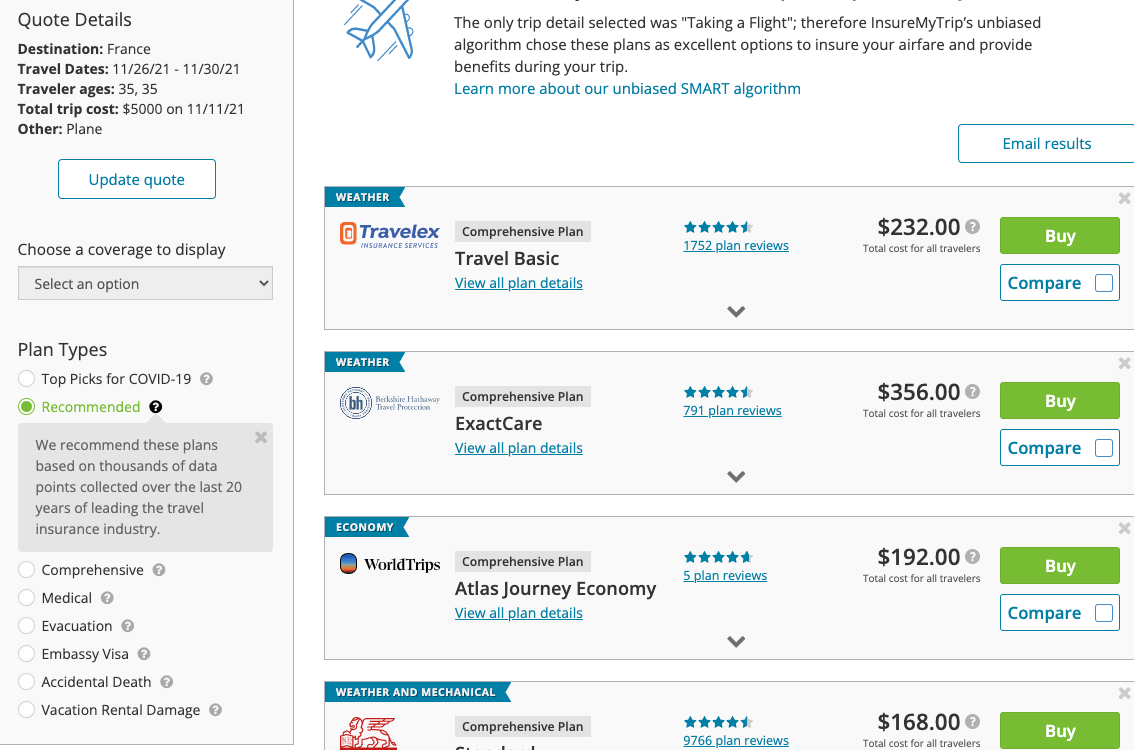**Detailed Descriptive Caption:**

The webpage is a quote details page for a travel company. It features a left-hand gray sidebar occupying one-quarter of the page, with "Quote Details" in bold black text at the top. Directly beneath, "Destination: France" is noted, where "Destination" is highlighted. Moving down, "Travel Dates" in bold marks the period from 11/26/21 to 11/30/21 in American date format. Then, "Traveler Ages" in bold highlights an age of 35. The "Total Trip Cost" is also boldly noted as $5,000, dated 11/11/21. "Other" is listed in bold, specifying "Plane" for travel mode. At the bottom, a white button with "Update Quote" in blue text is clickable. Below, a medium black font indicates the selection option area for coverage along with a gray button and a downward arrow. Also listed are various plan types, selectable via circles including "Top Picks for COVID-19" marked with a gray question-marked bubble, "Recommended" marked with a green bubble, and several other coverage options like "Comprehensive", "Medical", and "Evacuation".

The right three-quarters of the page is white, featuring the dorsal view of an airplane's outline in dark blue. Adjacent to this is text explaining "The only trip details selected was 'taking a flight'", justifying plan options provided by Ensure My Trip's algorithm. Below, a blue link "Learn more about our unbiased smart algorithm" provides further reading. A clickable white "Email Results" button in blue resides below this. Four plan fields in gray follow, each introducing travel plans with different details like plan names, prices, ratings, and actionable buttons.

- The first field starts with "Weather" in white on a blue button, an orange icon, a mention of "Travel X" and "Comprehensive Plan" in black on gray, and "Travel Basic" in medium font. It offers a view link, a star rating of 4.5 with 752 reviews, priced at $232.00. Buttons for buying and comparing options are present.
- The second field with an indistinguishable logo, starts similarly with "Comprehensive Plan" listed in black on gray, "Exact Care" in medium font, and a star rating of 4.5 with 791 reviews, priced at $356.00.
- The third has "Economy" on blue, a "World Trips" icon, and "Atlas Journey Economy" in black. It has five-stars but only five plan reviews, and is priced at $192.00.
- The fourth, partially shown, mentions "Weather and Mechanical" on blue, a red Griffin-like image, and a 4.5-star rating with 976 reviews, priced at $168.00.

Each of these plans also includes total cost information, green "Buy" buttons, blue "Compare" buttons, and 'X' icons for removal.